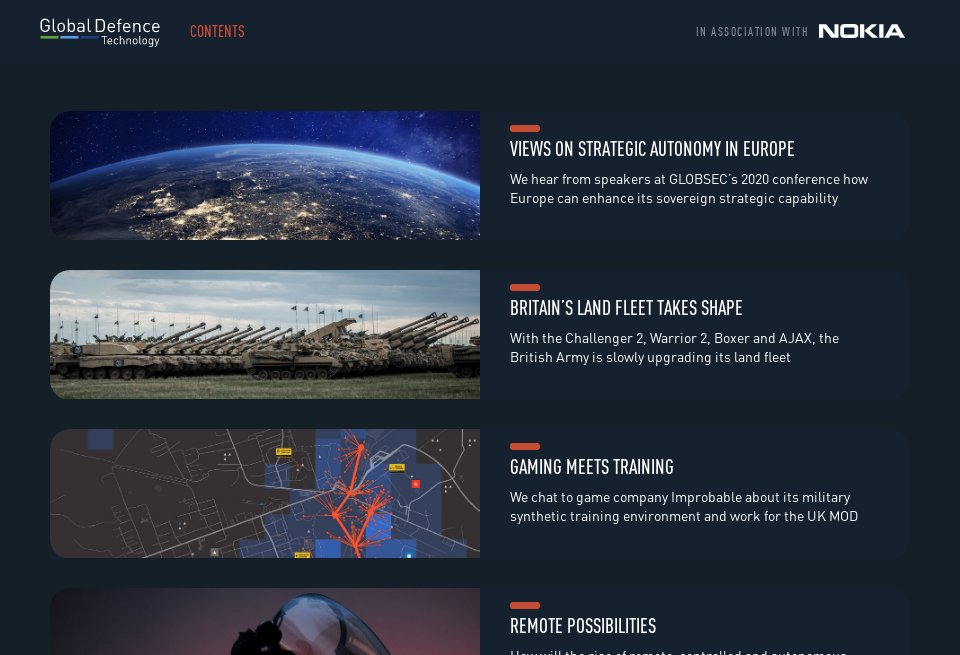In this visually arresting image, potentially a promotional poster or an advertisement, the background is stark black, lending an air of sophistication and gravity. Featured prominently in large white letters at the top left corner are the words "Global Defense Technology." Underneath "Global," two thin lines—one green, the other sky blue—add a touch of color. 

To the right of this main title, the word "Contents" appears in bold red. Further right, the statement "In association with Nokia" is prominently displayed, with "Nokia" emphasized in bold white font.

The left side of the image is segmented into a column of four rectangular images. Each image is accompanied by a brief descriptive headline and a line of text to its right in white, framed above by a thin red line:

1. **Top Image:** Depicting the curvature of the Earth as seen from space, it is tagged with the headline "Views on Strategic Autonomy in Europe."
   
2. **Second Image:** Featuring a lineup of gray tanks with their barrels pointed skyward, this image is labeled "Britain's Land Fleet Takes Shape."
   
3. **Third Image:** Showing a basic street map overlaid with red lines marked by small, explosive bullet points, it carries the title "Gaming Meets Training."

4. **Bottom Image:** Only half-visible, this image appears to show the top of a man's head. The headline beside it reads "Remote Possibilities."

Collectively, these elements create a captivating and structured visual narrative, emphasizing the multifaceted aspects of global defense technology while highlighting key topics in contemporary military and strategic discourse.